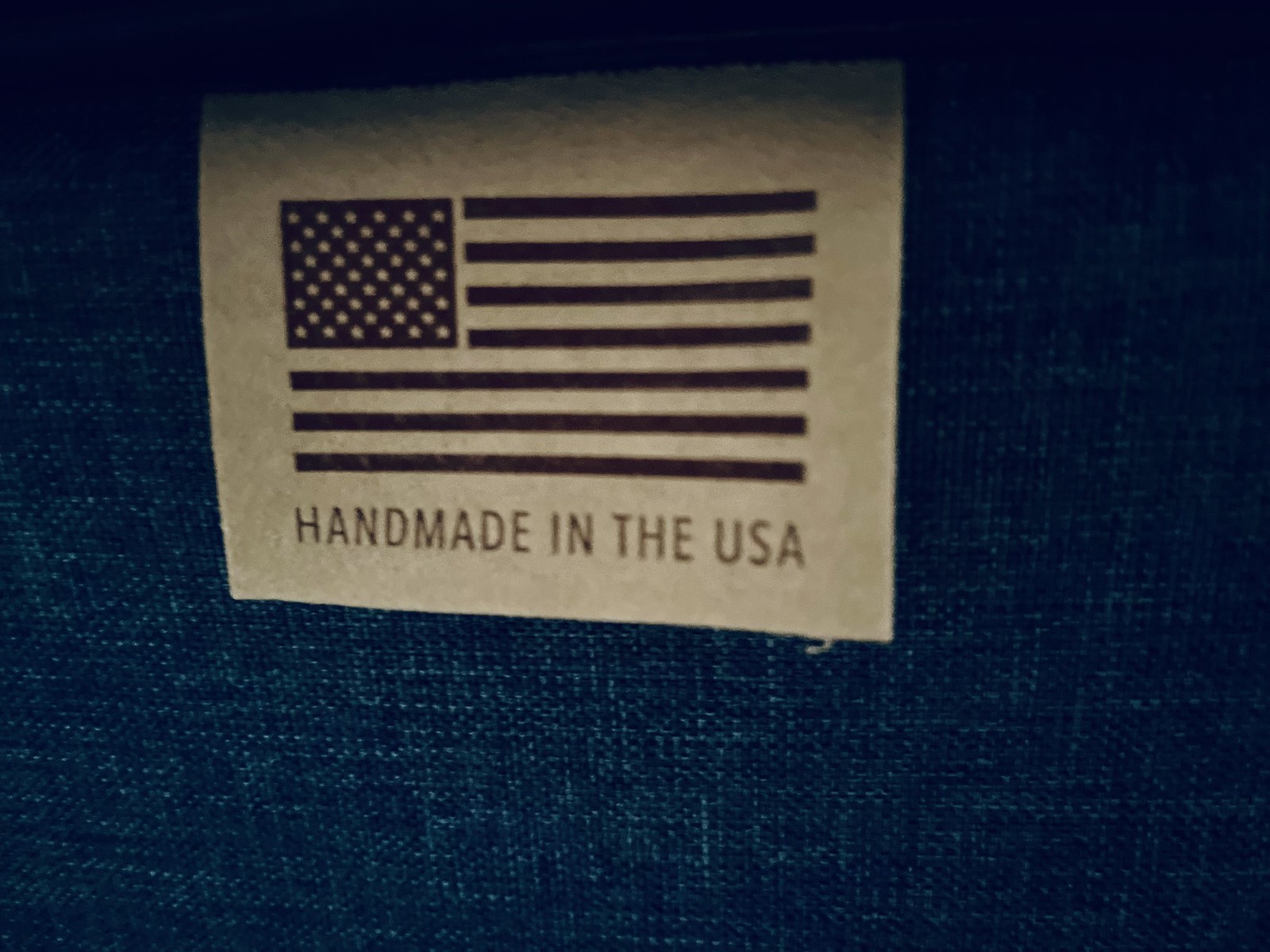The image features a detailed close-up of a dark blue denim fabric that serves as the background for the entire photo. Centered prominently on this dark denim is a square, off-white or cream-colored label. The label displays a stylized representation of the American flag at its center. The flag consists of simplified elements: seven stripes and a field of stars, where the stripes and the stars appear to share a similar color palette. The field of stars, possibly set against a dark blue background bordered in black, appears to have stars that are outlined in a black hue. Below the flag, the text "Handmade in the USA" is inscribed in a brown color, adding an artisanal touch to the garment label.